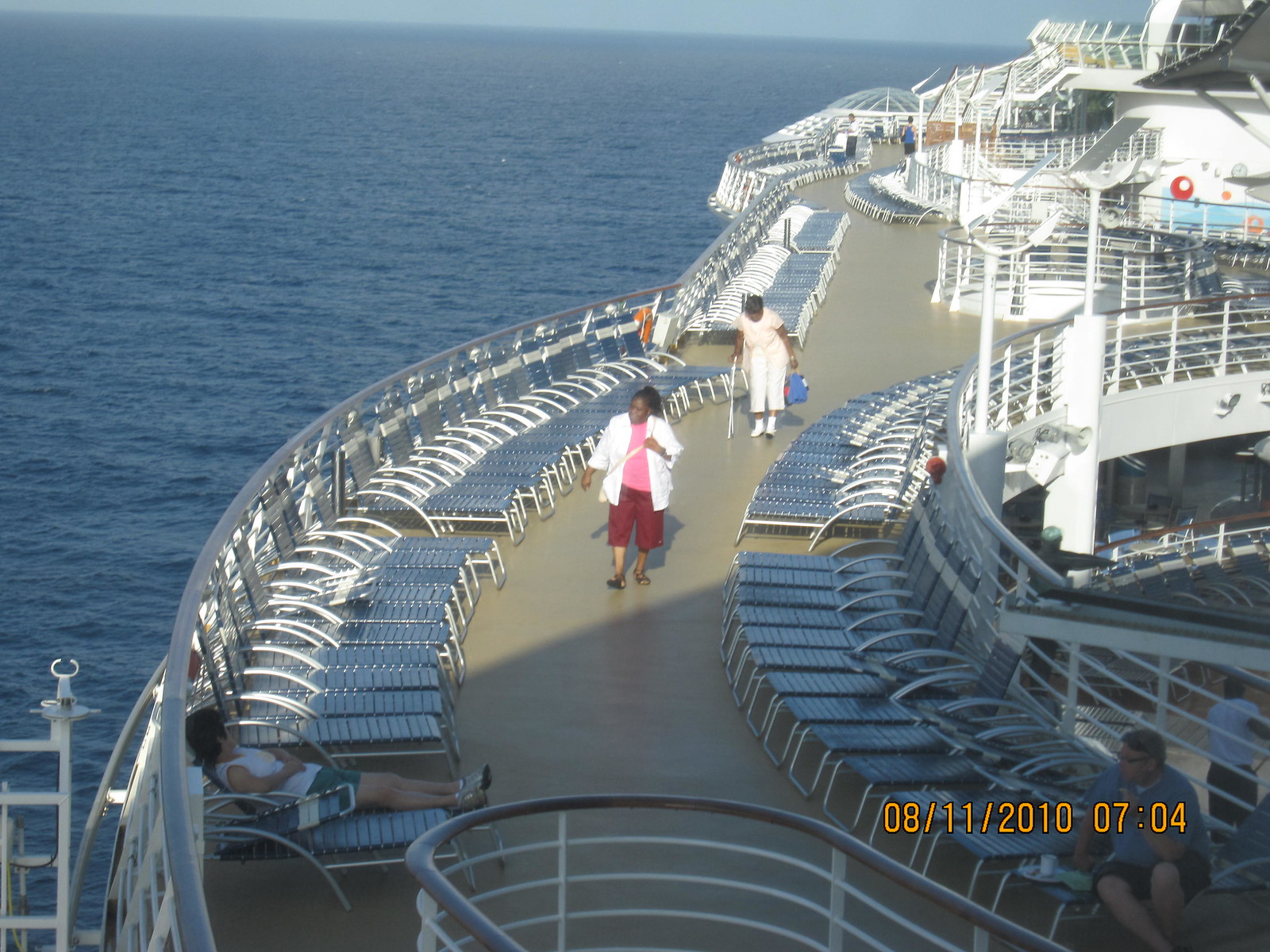In this vibrant color photograph taken on August 11, 2010, the expansive top deck of a cruise ship stretches out under a clear sky, bordered by the vast blue ocean occupying nearly half the frame. The tan-colored deck is partially populated, giving a sense of spaciousness. Lined with numerous beach and sun tanning chairs, the deck edges overlook the serene water. Close to the foreground, a man in a blue shirt and black shorts lounges on a deck chair with a tray holding a cup, possibly coffee or tea. Opposite him, a woman in a white shirt, blue shorts, and sneakers is similarly reclining. 

In the mid-ground, a woman dressed in red shorts, a pink shirt, and a white jacket strides toward the photographer, accompanied by another woman, possibly a woman of color, in white attire walking with a cane. Near them, a staff member in a whitish outfit methodically cleans up rubbish using a pole and bag. Background figures are dispersed across the deck, enhancing the sense of a leisurely yet lightly crowded environment. The deck's railings lead to various double-height spaces and staircases, contributing to the sprawling and multi-leveled layout of the ship's amenities.